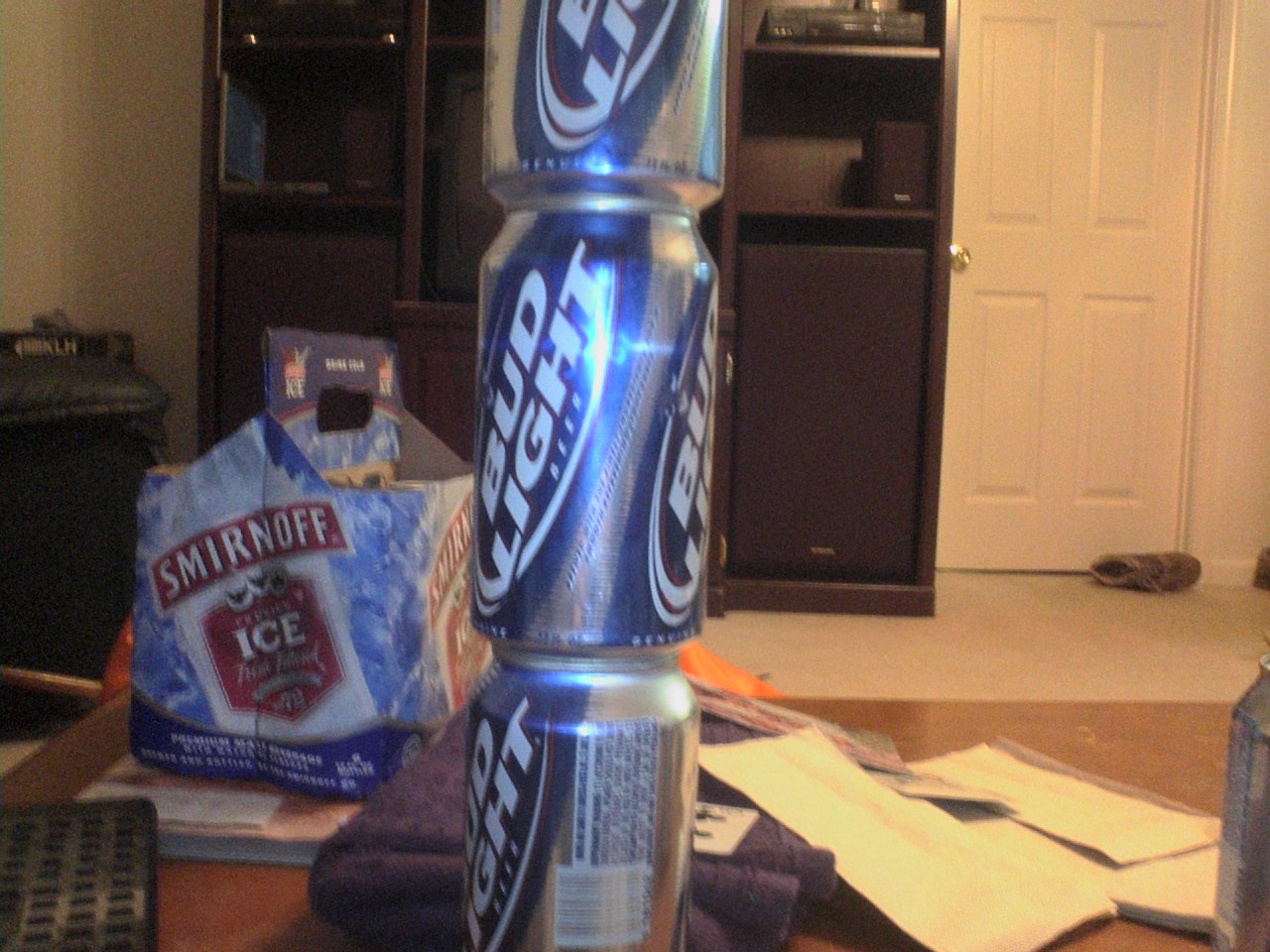This interior photograph, likely taken in a living room of a house or apartment, features a cluttered yet realistically lived-in setting. The background presents a tan-colored wall with a matching door that has a silver doorknob. On the floor near the door, a sneaker is visible. Adjacent to this, there is a dark wood entertainment center equipped with several shelves, housing a TV that is partially obscured by the main subject of the image - three vertically stacked Bud Light beer cans in blue and silver, emblazoned with white diagonal text reading "Bud Light".

In the foreground, a lighter wood coffee table displays an array of items, contributing to a sense of casual disarray. On the table, there are opened white envelopes scattered about, possibly bills, alongside a dark and dirty TV remote control. A cardboard container for Smirnoff Ice, bearing a handle and logo but without any bottles inside, sits prominently. Under this container, there appears to be a blue folded cloth and perhaps a book. The overall composition reveals a snapshot of everyday life, with entertainment and refreshment juxtaposed against a backdrop of ordinary household clutter.